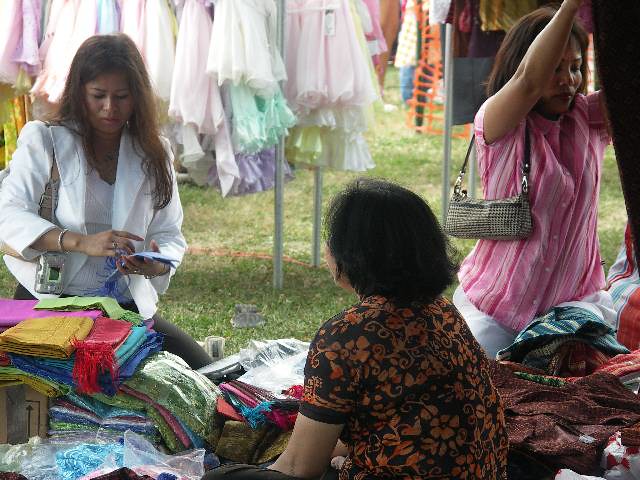The image depicts an outdoor flea market scene set on a flat, grassy area under broad daylight. At the center of the image, three women are engaged in shopping activities. In the foreground, one woman sits on a blanket laden with clothes, appearing to inspect various fabrics and garments. She wears a black shirt adorned with floral patterns. On the right, another woman kneels and examines a piece of blue fabric, dressed in a white shirt paired with a white overcoat. She has long brown hair and a camera by her side. On the left, a third woman is lifting a piece of fabric above her head, dressed in a pink shirt with a purse slung over her right shoulder, as she evaluates the clothes. Surrounding them are piles of various fabrics and garments, including shirts and dresses. In the background, racks full of hanging clothes, such as dresses, further set the market scene. The vivid tapestry of colors in the image includes pink, white, blue, green, purple, black, different shades of red, gray, and orange. The entire setting conveys a lively market atmosphere with no visible text.